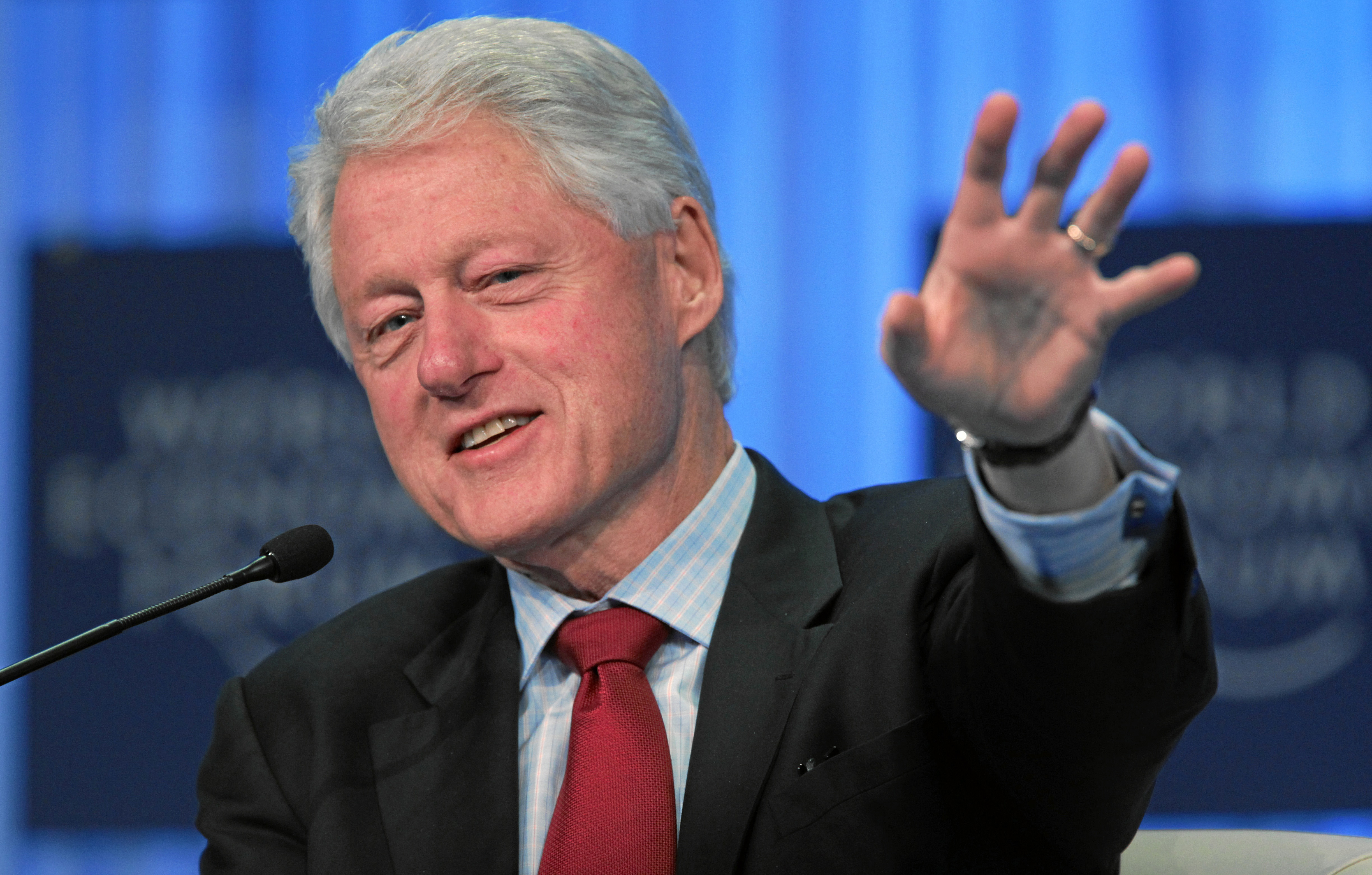In this image, former U.S. President Bill Clinton is the focal point, positioned primarily in the center. He is captured mid-speech, smiling, with his mouth open and teeth visible, looking slightly off to the center of the image. Clinton, a Caucasian man with a slightly reddish hue to his skin, has well-groomed white and gray hair with some wrinkles visible near his eyes. He is dressed in a black suit jacket, paired with a light blue and white button-up shirt and a burgundy red tie. His left hand is raised, displaying a wedding ring and a watch, possibly in a waving gesture or mid-motion during his speech. In front of Clinton, emanating from the bottom left corner of the image, stands a small black microphone on a stand.

The background appears to be indoors, characterized by light blue curtains that span most of the image and form the backdrop for the scene. These curtains are slightly out of focus, adding a soft blur that creates depth. Flanking the curtains are two dark blue square signs or posters, one on the left and one on the right of the background. These posters contain some white text, but the blur renders the details unreadable. The overall color palette of the image includes light blue, dark blue, black, white, red, tan, and gray, adding to the formality of the setting, which appears to be a speech or public address.